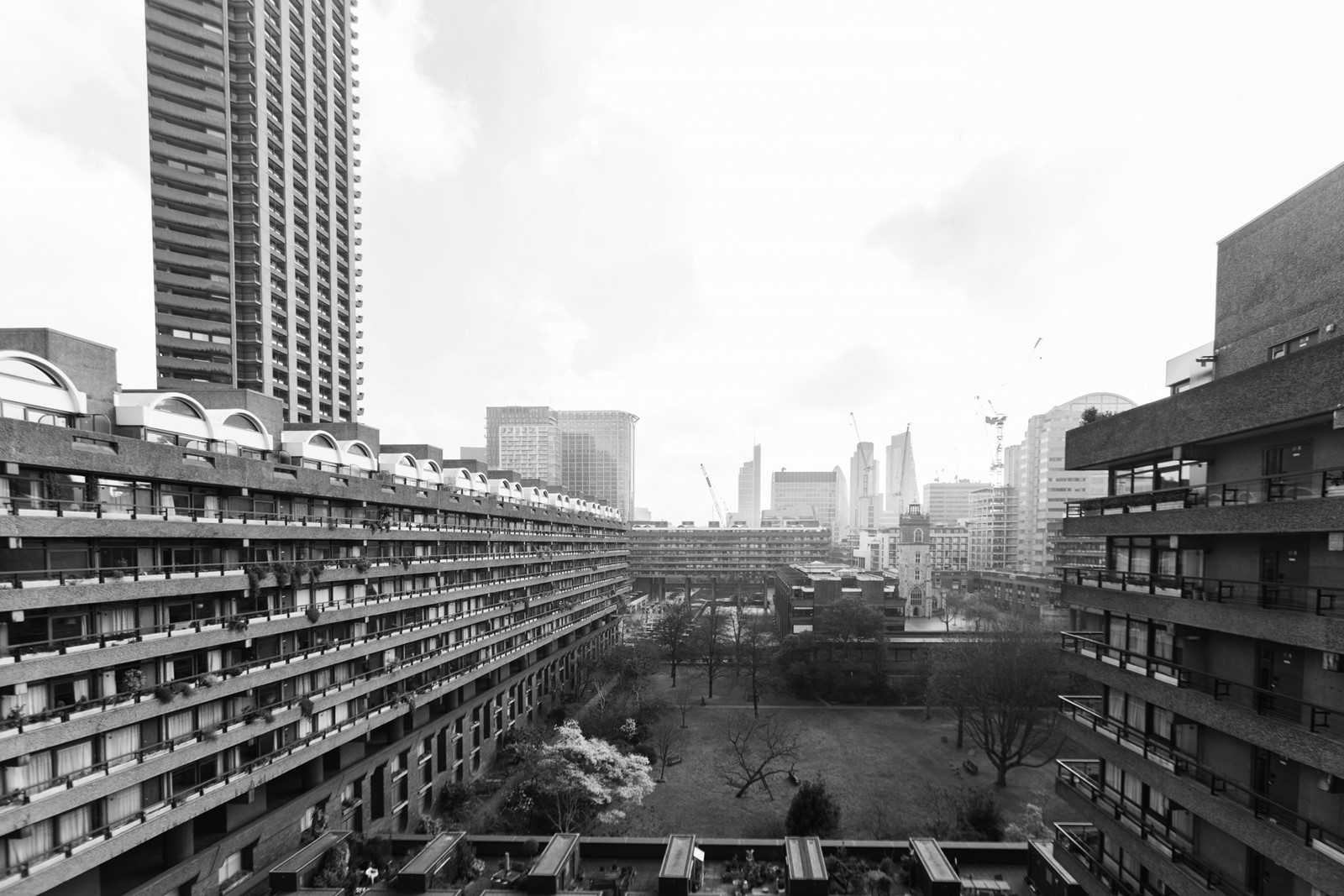This black and white photograph, likely taken in the 60s or 70s, showcases an industrial or perhaps low-rent residential area under a gloomy, overcast sky. The composition is framed by two multi-story buildings on either side, with visible balconies and windows. The building on the left features a couple of stories, and round-shaped windows at the top, with some plants growing on its walls. To the left of this building, an imposing skyscraper stretches upwards, its top cut off by the image's edge. On the right side, another multi-story building with a flat rooftop mirrors the one on the left but appears shorter and less imposing. Both buildings are set along a perspective that points towards the middle of the frame, where the distant city skyline rises. The background is filled with additional skyscrapers, blurred through the foggy atmosphere. Along the bottom of the photograph, there is a hint of a park area with trees and flat ground, indicating a touch of greenery in the otherwise heavily built-up scene.